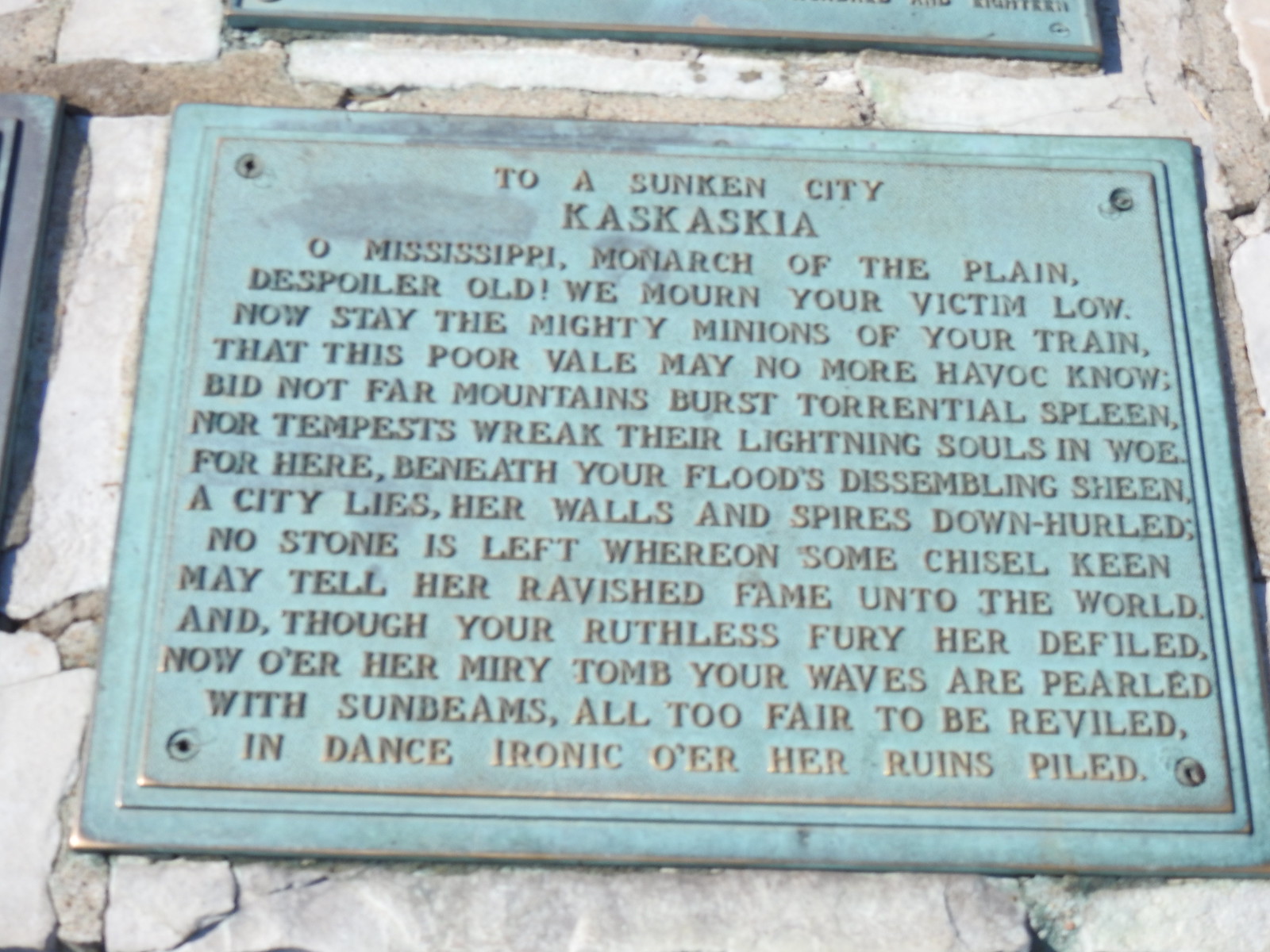The image depicts a plaque mounted on a gray stone or cement wall, secured with four bolts at its corners. The plaque is primarily a greenish-gold color, heavily weathered and rusted, which gives it a mostly green appearance. The background of the plaque is a pale light blue, featuring accents of gold and copper. The plaque bears the text of a poem dedicated to a sunken city, Kaskaskia. The poem reads: 

"To a sunken city, Kaskaskia. Oh Mississippi, monarch of the plain, despoiler old, we mourn your victim low. Now stay the mighty minions of your train, that this poor vale may no more havoc know. Bid not far mountains burst torrential spleen, nor tempests wreck their lightning souls in woe. For here beneath your floods' dissembling sheen, a city lies, her walls and spires down hurled. No stone is left where on some chisel keen may tell her ravished fame unto the world. And though your ruthless fury her defiled, now o'er her miry tomb your waves are pearled with sunbeams all too fair to be reviled, in dance ironic o'er her ruins piled."